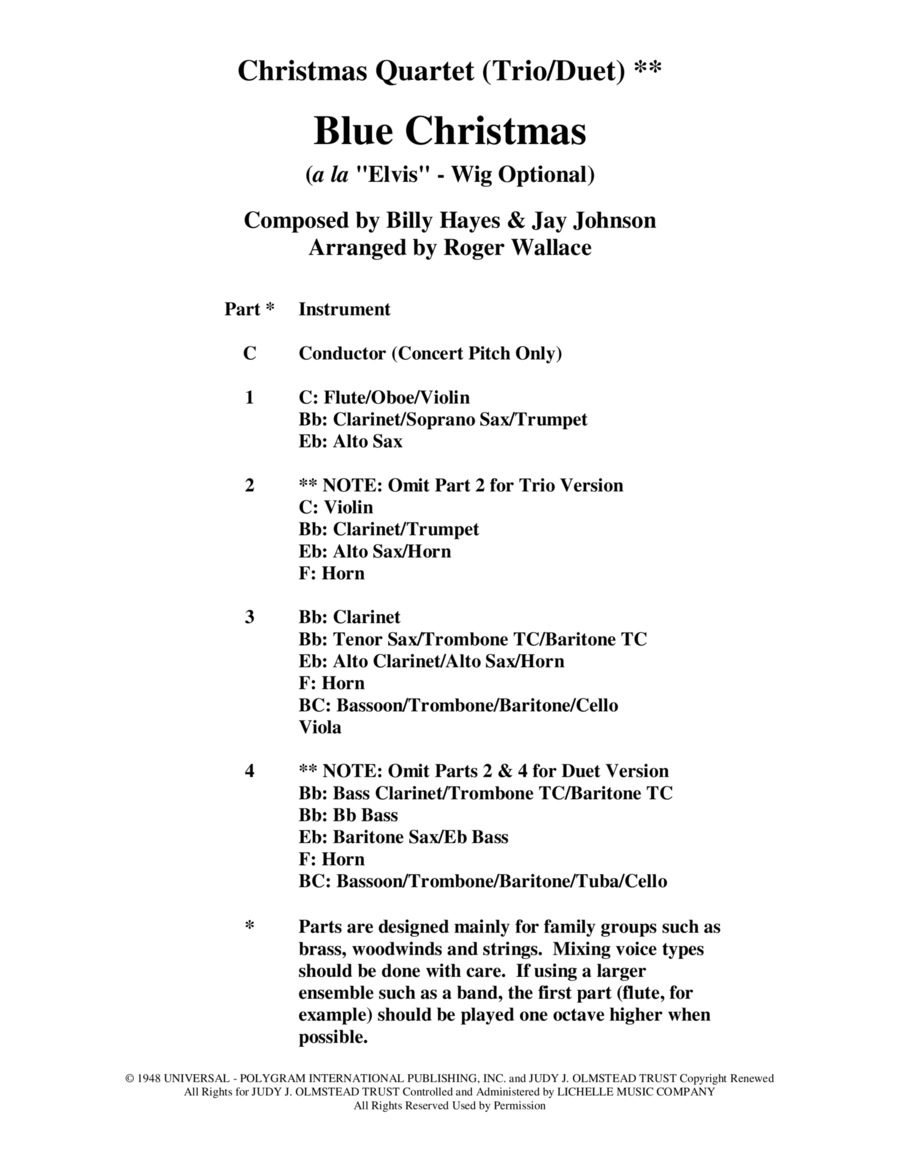The image consists of a white background adorned with black text, likely extracted from a book or website. At the top, the title reads "Christmas Quartet (Trio/Duet)" accompanied by two asterisks. Directly beneath it, in the largest and most bold font, is the title "Blue Christmas," followed by the note "a la Elvis - wig optional." The song is composed by Billy Hayes and Jay Johnson, and arranged by Roger Wallace. The document lists details regarding musical parts and instruments, indicating a setup for various configurations such as quartets, trios, or duets. It specifies sections labeled as Part C (Conductor), 1 (Flute, Oboe, Violin), 2 (Violin, Clarinet, Trumpet, Tenor Sax, Horn), 3 (Clarinet, Sax, Horn), and 4 (same as Part 3). The arrangement aims at family groupings of brass, woodwinds, and strings, with a note advising that larger ensembles, like bands, should have the flute part played one octave higher when feasible. At the bottom, minimal but important copyright information is printed, stating "1948 Universal, Polygram, International Publishing Inc." along with some additional credits.